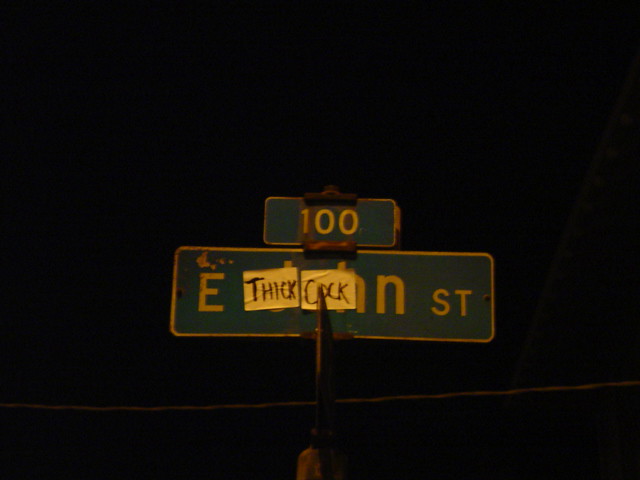A nighttime photograph captures a defaced street sign against a pitch-black background, emphasizing the altered sign as the sole focus. The sign, illuminated against the surrounding darkness, features the traditional green rectangular shape with rounded corners. At the top, the number "100" stands out in stark white lettering. Below the number, the sign originally indicated "East John Street." However, the word "John" has been obscured and defaced with two pieces of white tape. On the tape, the words "Thick Cock" are handwritten, effectively altering the original street name with the visible, crude message adhered to the street sign. This act of vandalism stands out prominently against the night, captured crisply by the camera.